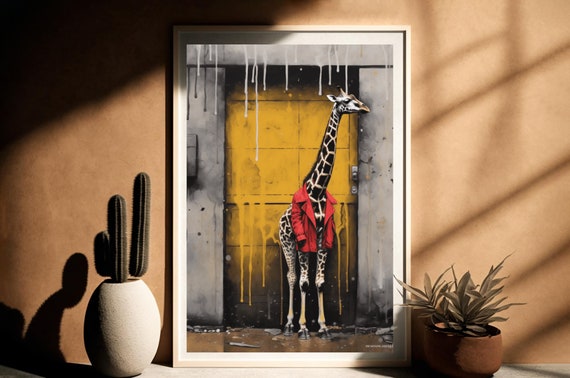The photograph captures a painting of a giraffe set against a peachish-pink adobe wall with considerable natural light streaming in from the right, creating intriguing play of shadows. To the left of the painting is an oval-shaped white vase containing two cacti, positioned on a gray table or ground. The cactus on the right is slightly taller than the one on the left. To the right of the painting stands a brown vase filled with green foliage.

The painting itself, leaning against the wall, is framed with a sequence of a thin white strip, a thick black strip, and then an even thicker white strip. It depicts a black and white giraffe donning a red coat, standing in front of a surreal, melting mustard-yellow door with a gray frame, giving it an abstract, dreamlike appearance. The giraffe's head is slightly turned to the right, and its legs exhibit a gradient from black and white to entirely white from the knees down, suggesting an impossibility that hints at AI-generated art.